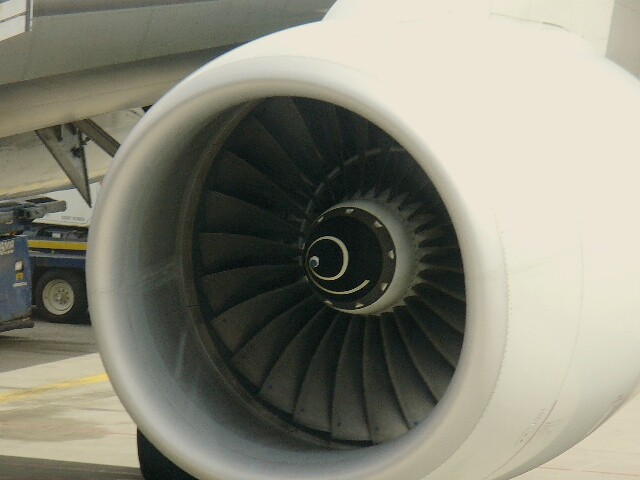The image depicts a close-up view of a commercial airliner’s jet engine, prominently featuring the large, round, white engine housing suspended from the wing, although the exact attachment is partially cut off at the top edge of the image. The engine's interior showcases an array of dark, slightly curving fan blades with a central hub in the middle, holding them in place, surrounded by smaller bolts. The fan blades appear distinct and still, indicating that the engine is not currently in operation. The engine dominates the frame, with a faint glimpse of the aircraft wing connecting to it at the top.

On the bottom left side of the frame, partly obscured by the engine, a blue vehicle - likely used for baggage handling or airport ground services - is visible. Only the back wheel and part of its flatbed can be seen. The vehicle's body appears to have a blend of blue and gray colors. In the lower right corner and extending toward the left, there is pavement marked with a yellow line.

Overall, the scene captures the jet engine in pristine, well-maintained condition under daylight, with some surrounding elements hinting at the bustling environment of an airport tarmac.